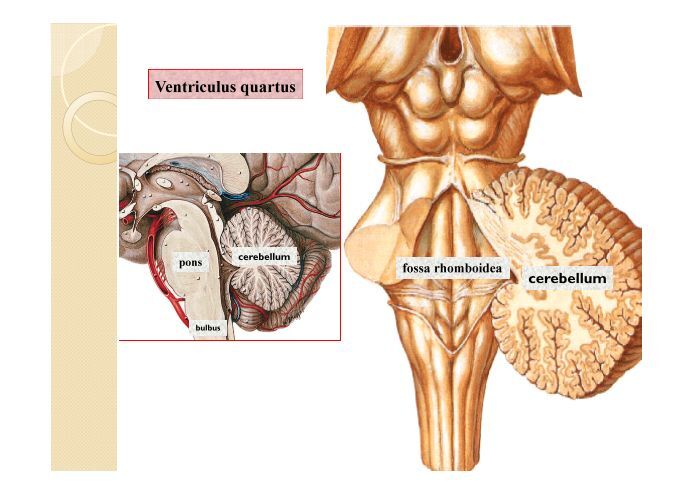This image is a detailed medical drawing, potentially from a biology or medical textbook, illustrating several anatomical components with a focus on the brain and related structures. Dominating the left side of the artwork is a labeled horizontal rectangle with "ventriculocortis" in red text. Adjacent to it is a gold bar overlaid with incomplete thin and thick circles ending at the bar's edge.

At the bottom part of the image, there's a depiction of the lower brain and the upper neck region. Specifically, on the left side of the neck's front is an off-white section, likely depicting part of the nervous system, with a prominent vein running in front of it. Labels indicate the "pons" near the Adam's apple area and "bulbous" further down.

On the right-hand side, the cerebellum is prominently displayed with intricate detailing. The image highlights the bottom part of the brain, showing a blood vessel extending into it, and outlines layered skin and cartilage beneath the cerebellum. Moreover, there is a detailed dissection of the cerebellum represented in a bronze color, revealing the internal brain matter. Another section, labeled "fossa rhomboidea," depicts the stalk leading to the cerebellum, which is depicted halved to show its inner structure.

The overall color scheme includes dark skin tones and orange hues, enhancing the educational and scientific feel typical of textbook illustrations.